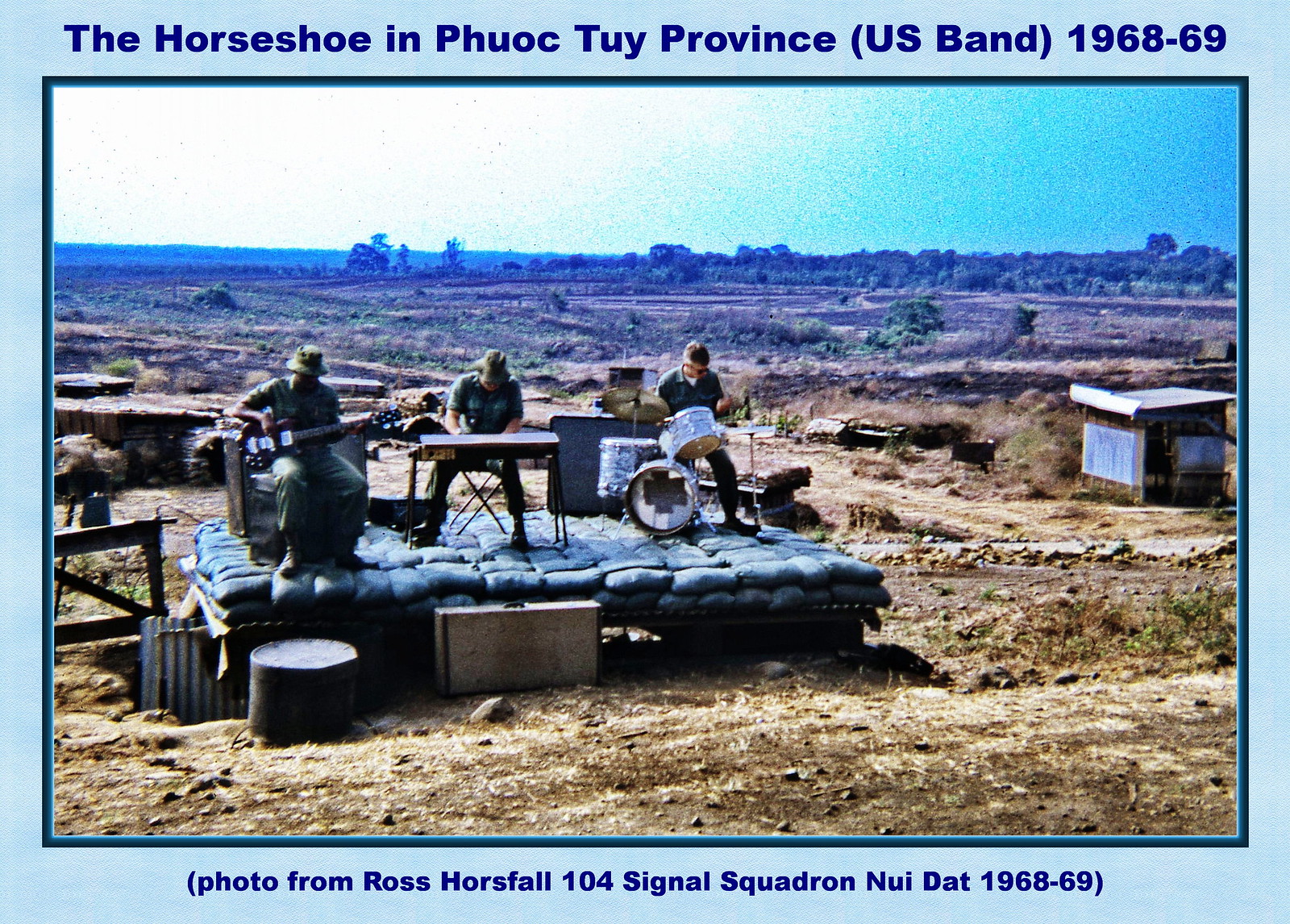The photograph features a U.S. band performing on a makeshift concert stage constructed from sandbags in the middle of a desert-like environment. Three musicians are present: a guitarist on the left, a keyboard player in the center, and a drummer on the right. The scene is set against a backdrop of sparse trees and dirt, with a small metal shed visible on the right side. The image is bordered with a light blue frame, and at the top, in dark blue text, it reads, "The Horseshoe in Phuoc Tuy Province (U.S. Band 1968 to '69)." At the very bottom, another caption states, "(Photo from Ross Horsefall, 104 Signal Squadron, Nui Dat. 1968 to '69)."